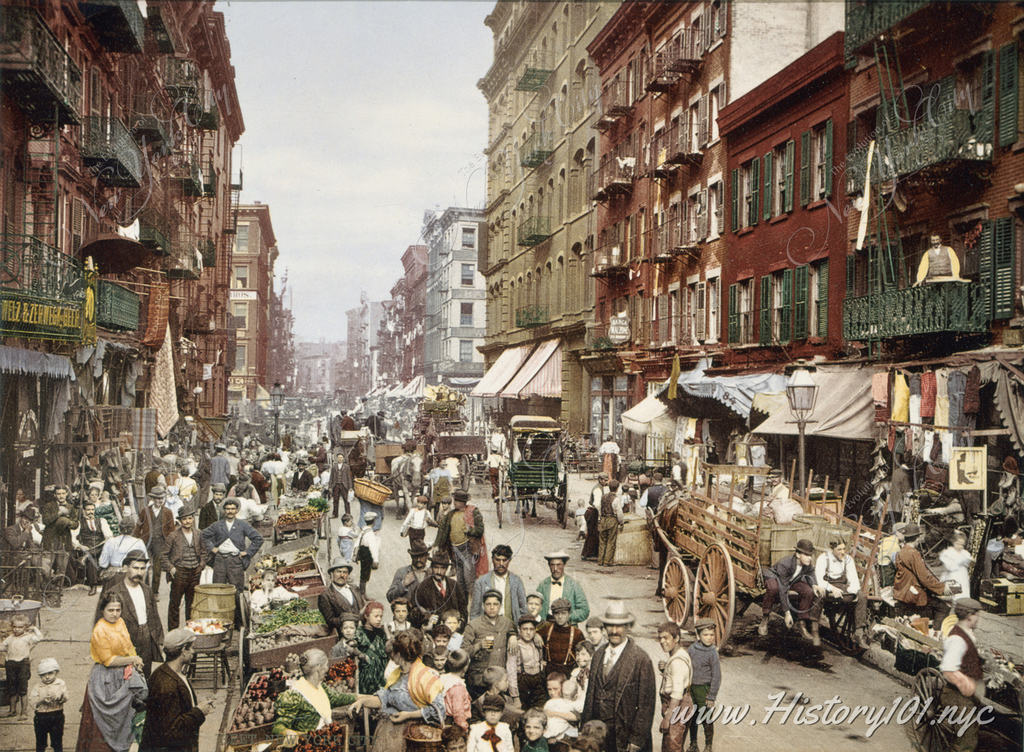The vibrant scene captured in this colorized vintage photograph depicts a bustling market street in an old New York City neighborhood. Large multi-story buildings, painted in shades of brown and red, line either side of the busy street, with laundry hanging from their balconies. Street lamps and various amenities dot the thoroughfare, enhancing the historical charm of the setting. In the center of the image, a large wooden cart, drawn by a black horse, holds men, who appear to be vendors or customers, seated in the back. The street is alive with activity; men, women, and children are gathered, some huddling together while others peruse the numerous vegetable stalls selling fresh produce, including potatoes and carrots. The atmosphere is one of organized chaos, a hallmark of urban market life in a bygone era. A white watermark reading "www.history101.nyc" is visible in the lower right corner, grounding the image in its historical context.